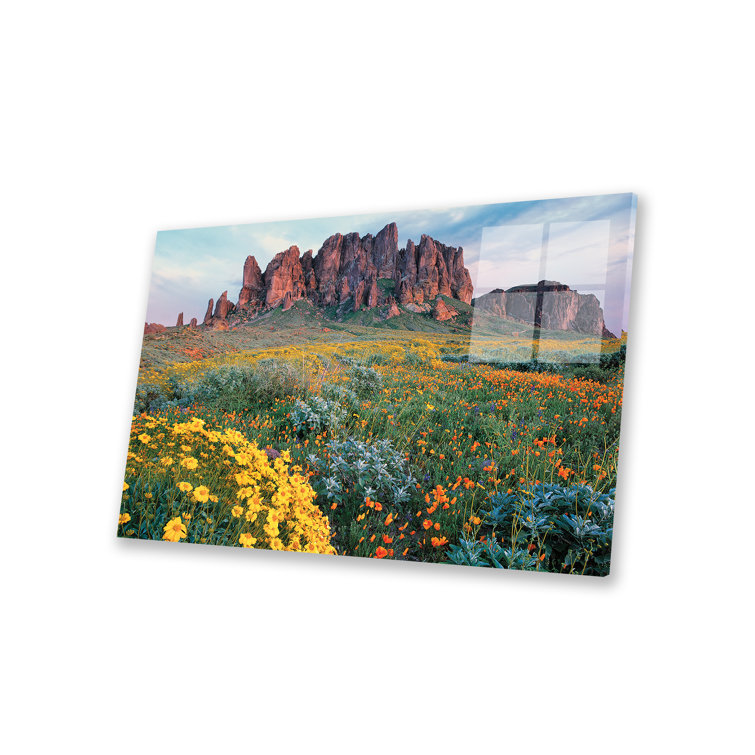The image depicts a realistic photograph, possibly a canvas art piece, showcasing an expansive and colorful natural landscape. Dominating the scene is a large, jagged rock formation with a reddish hue, featuring darker areas in the middle. This formation is set against a backdrop of a blue sky interspersed with white clouds. In front of the rocks lies a vibrant field bursting with wildflowers of various colors, including bright yellow, blue, orange, red, and purple. Closer to the rock formation, the wildflower field transitions into green grass. In the top right corner of the image, the Windows logo is prominently displayed, appearing as a large white square divided into four smaller squares by a cross-like structure, subtly blending into the scene. The photograph was taken during the day, evident from the clear and well-lit quality of the entire landscape. There are no animals, people, or other living creatures present in the image.